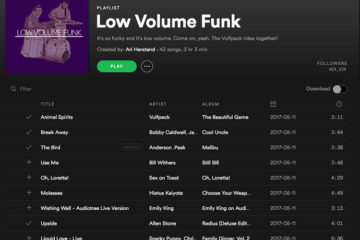This image falls under the category of websites. The webpage features an all-black background with extremely tiny text, making it difficult to read or enlarge. At the top, there is a green "Play" button situated in the right-hand corner, directly above the phrase "Low Volume Funk" written in white letters. Below this header, a purple box contains an image of two individuals, who might be musicians, though their actions are unclear due to the small size of the image. The central part of the page hosts a playlist, but the specifics of each track are largely illegible. Various buttons are visible: one appears to be a "Download" button, and another is a play button accompanied by a button with three dots. Partial track names such as "Animal Something," "The Bird," and "Upside" are barely discernible but suggest funk music content.